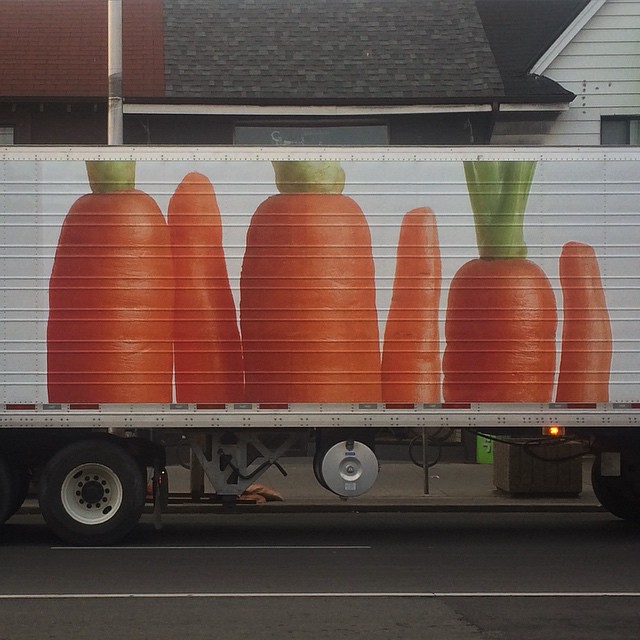This detailed photograph captures the side of a large 16 or 18-wheeler truck, specifically highlighting the vibrant and colorful advertisement on its side. The truck is driving down an asphalt road marked with white lines along the center and edge. The truck's base color is white with silver ridges aligning the top and bottom edges. Dominating the side of the truck is a brightly painted, detailed image of carrots. These carrots are depicted as partial images, alternating between the tops and bottoms, displayed side by side in a repetitive sequence of six, emphasizing their striking orange color and vivid green tops. The setting includes a building with a tiled roof, a white pole, and a white house to the right, contributing to a suburban backdrop. The image is clear and detailed, making it an effective advertisement likely intended to attract attention to a vegetable brand.